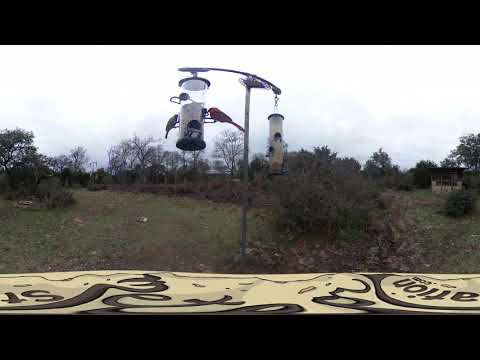The image displays a small grassy hill scattered with brown leaves. The overcast sky has a grayish hue, adding to the overall gloomy feel of the day. Central to the image is a gray metal pole fashioned in the shape of a 'T,' from which two bird feeders hang. One of these feeders houses a distinct red cardinal, while a few other birds are seen perching and eating. In the background, sparse trees with bare branches and partially filled bushes emphasize the autumn setting. Framing the scene from below is a brown bench with black writing, possibly distorted. To the right, more of the expansive yard is visible, featuring a structure that appears to be a brown shed. The entire setting evokes a tranquil yet somber mood typical of fall, on a cloudy day.